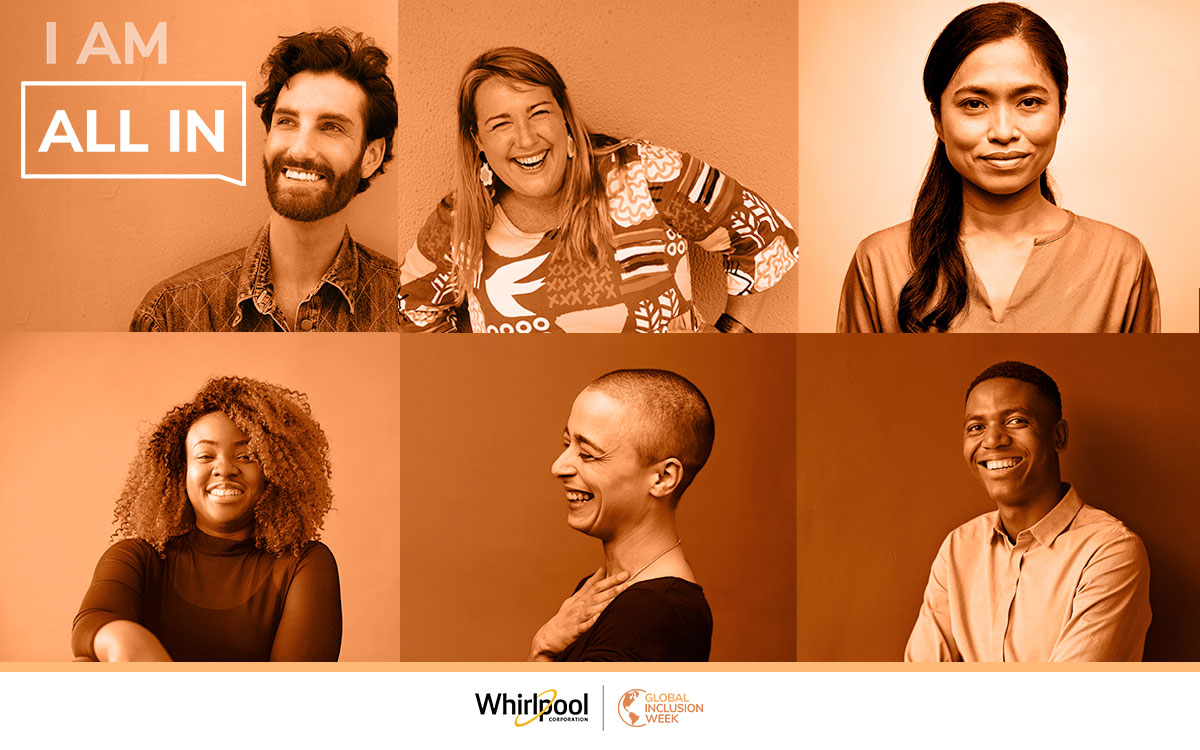This image comprises six sepia-toned portrait photographs arranged in a 3x2 grid. In the top left corner, the text "I am" appears followed by a speech bubble that says "all in." 

The top row features three portraits:
1. On the left, there is a white man with a beard and mustache, wearing a denim shirt, positioned towards the bottom left of the frame.
2. In the center, a white woman with blonde hair is captured laughing with a bright smile, hands on her hips, sporting a vibrant, funky shirt.
3. On the right, a straight-faced Asian woman with long black hair draped over her right shoulder is shown.

The bottom row contains the following portraits:
1. On the left, an African American woman with blondish, frizzy hair is facing the center while looking directly into the camera.
2. The center features another woman laughing, with her right hand placed on her chest. She is bald, wearing a black shirt and a necklace.
3. On the right, an African American man dressed in a button-up white shirt completes the grid.

All images share a uniform sepia tone that gives the collection a cohesive, warm, and slightly nostalgic feel.